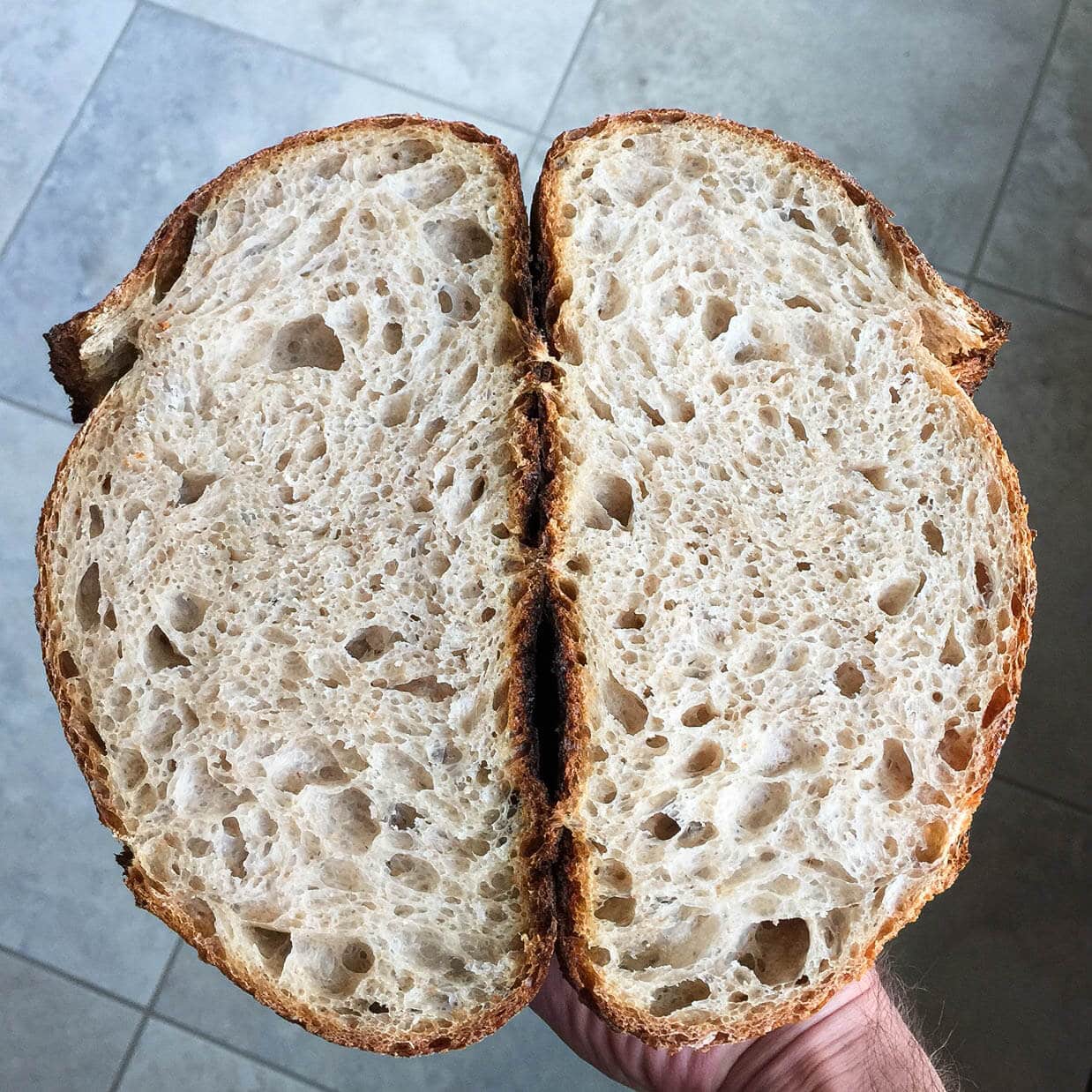The photograph, taken from a top angle indoors, captures a hand holding a large loaf of sourdough bread that has been cut in half. The bread, exhibiting a bright and dark brown crust, reveals a light and airy interior filled with numerous air pockets formed by gas bubbles from yeast fermentation. This burst of gas helps the bread rise during baking, contributing to its poofy texture. The hand, belonging to a Caucasian male with noticeable brown hair on his wrist, holds the bread over a background of large, blotchy gray tiles. Interestingly, the shape of the bread halves resembles a laying bunny rabbit, with the elevated crust parts mimicking the nose and ears, and the rounded back completing the image. The inside of the bread is creamy in color, accentuated by the plethora of airy holes.